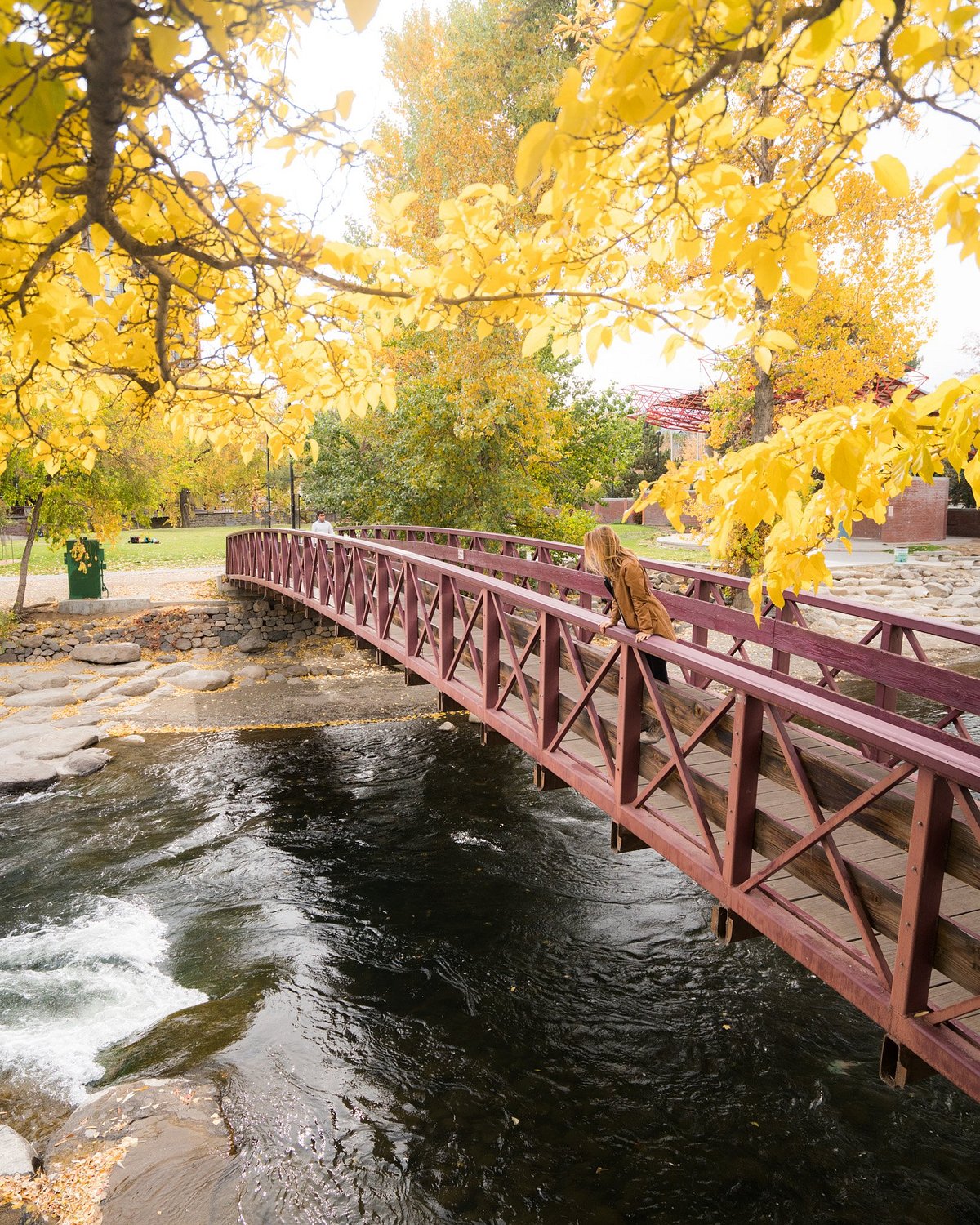The photograph captures a tranquil scene within a park, featuring a murky, dark green body of water, possibly a river or pond, flowing over granite rocks and creating slight rapids. A long, arched, burgundy-colored bridge made of wood and metal stretches across the water, with its closest end to the right of the image and extending to the left. Standing in the middle of this covered footbridge is a young woman with blonde hair, wearing a tan blazer, gazing thoughtfully into the water below. Beside her, a young man approaches, accompanied by a child. The bridge leads to a well-lit grassy walkway, hinting at a field in the distance. The setting is bathed in autumn's glow, with trees overhead displaying vibrant yellow leaves, while those in the background remain green. A large building, similar in color to the bridge, looms in the background, possibly part of the park's amenities. The scene is well-lit, suggesting a sunny, though slightly overcast day.